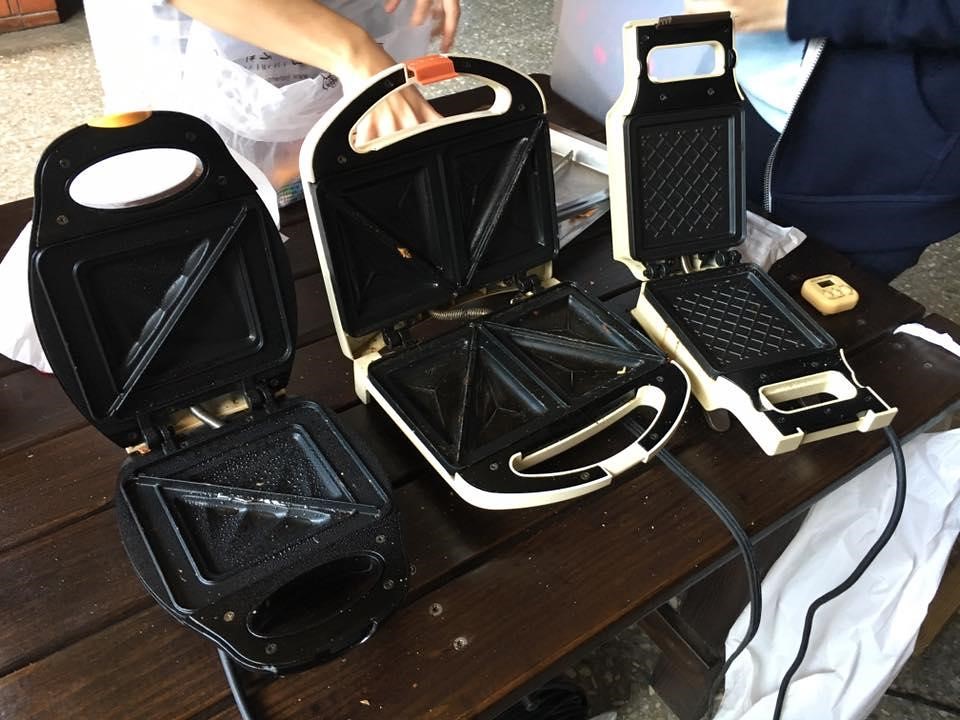This photograph displays three different waffle makers positioned side by side on a dark brown slatted wooden table. The first, an all-black waffle maker with an orange release button on the front handle, creates square waffles cut diagonally into triangles. The second waffle maker, which is white with black grilling surfaces and an orange clasp at the handle, produces two waffles or sandwiches, similarly shaped into triangles. The third and smallest waffle maker, also with a white exterior and black grilling surfaces, makes a single rectangular waffle. All three waffle makers are of clamshell design and visibly used, with traces of oil on their surfaces. Each is plugged in, with black cords trailing from them, and they sit open, revealing their interiors.

Behind the waffle makers, part of a person is visible, including their waist, part of their arm, and a hand reaching into a silver tray next to a white bag taped to the table for debris collection. Another person, dressed in a navy blue sweatshirt and blue shirt, stands at the far right side, partially visible at the end of the table. To the right of the smallest waffle maker is a small yellow hand timer, presumably for timing the cooking process. Additionally, in the upper right corner of the image, a large chrome container or possible freezer, partially off-screen, can be seen holding ingredients.